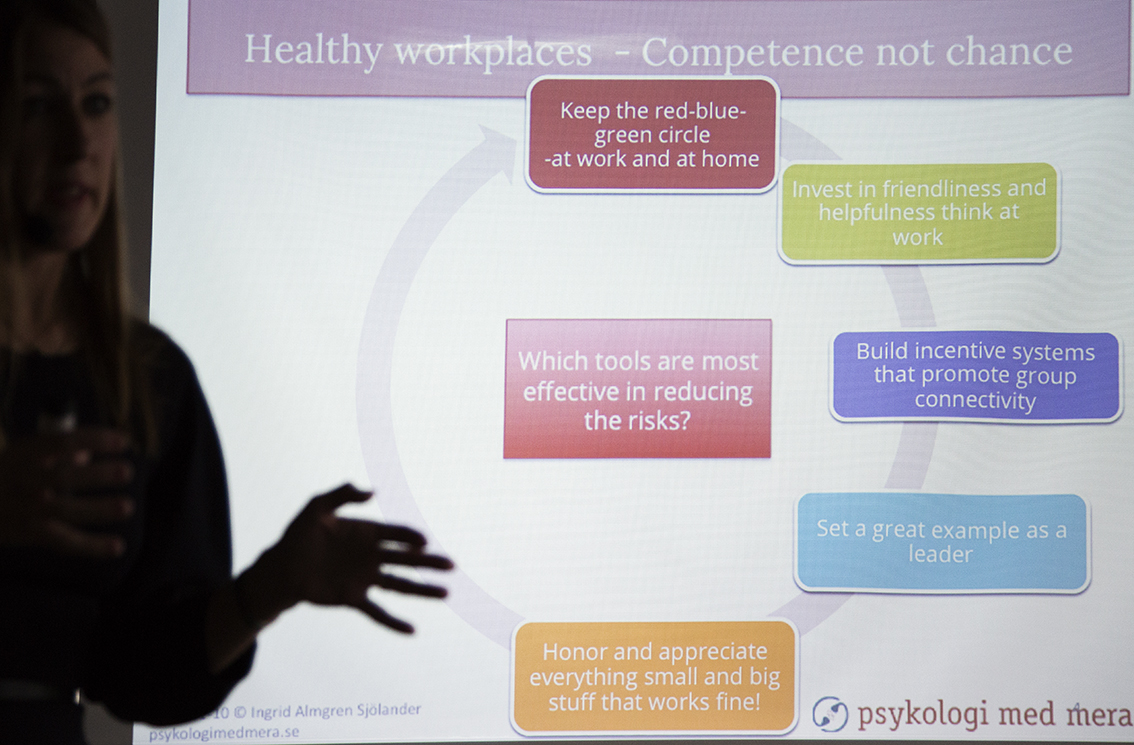In this photograph of a business meeting, a Caucasian woman with long, dirty blonde hair stands at the edge of the image, presenting a PowerPoint slide that takes up the majority of the photo. She is behind a projection screen displaying a graph titled "Healthy Workplaces, Competence, Not Chance." The slide features various colored boxes with text revolving in a circular arrow, pinpointing strategies to enhance workplace efficiency and safety.

Highlighted boxes include:
- A red box stating "Keep the red, blue, green circle at work and at home."
- A green rectangle advising, "Invest in friendliness and helpfulness; think at work."
- Another red box asking, "Which tools are most effective in reducing risks?"
- A blue box encouraging the building of "incentive systems that promote group connectivity."
- A light blue box recommending to "set a great example as a leader."
- An orange box urging to "honor and appreciate everything small and big that works fine."

The woman's hand is partially illuminated by the light from the projector, giving it a shadowy, skeletal appearance while she points to the slide. Overall, the image captures a detailed scene of an educational session focused on strategies for cultivating healthy workplace environments.